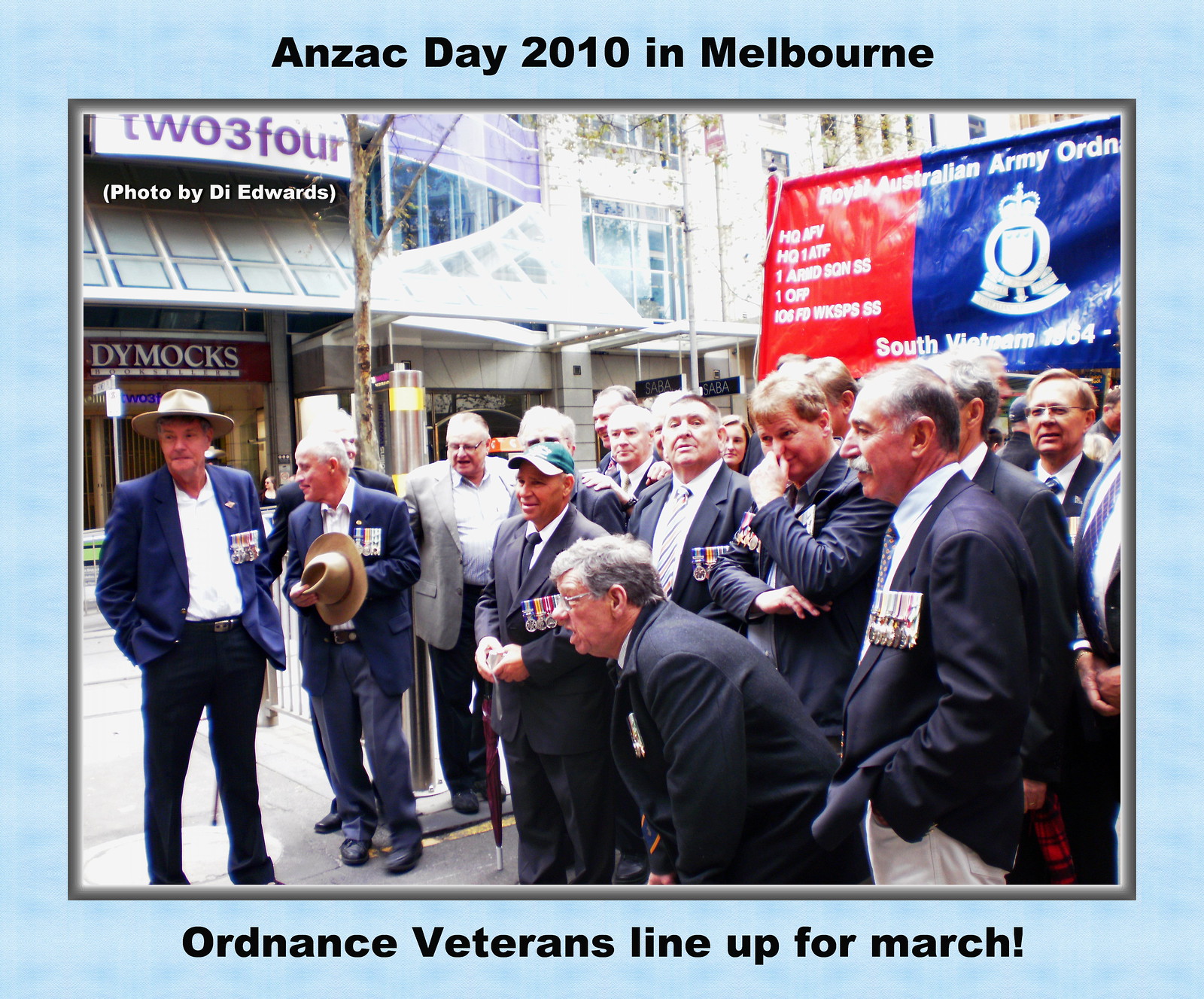The image depicts an outdoor scene in a city street, likely Melbourne, during a daylight celebration. It is framed by a light blue border, resembling a sky with scattered white clouds, with text at the top reading "Anzac Day 2010 in Melbourne" and at the bottom stating "Ordinance Veterans Line Up for March." Central to the photograph is a large group of older men, mostly in their late 40s to early 70s, predominantly with gray hair and dressed in dark blue blazers adorned with numerous medals on their left breast pockets. The men are positioned towards the center, though they are primarily looking to their left, suggesting they are preparing for another photograph. Behind them, a large red and blue banner with the crest of the Royal Australian Army is partially visible, along with text that includes "Royal Australian Army" and obscured references to "South Vietnam 1964." The background also showcases distant buildings and city street elements, contributing to the parade-like atmosphere. Additional text from the photographer, "photo by D. Edwards," appears in the photo, indicating the author of the image.